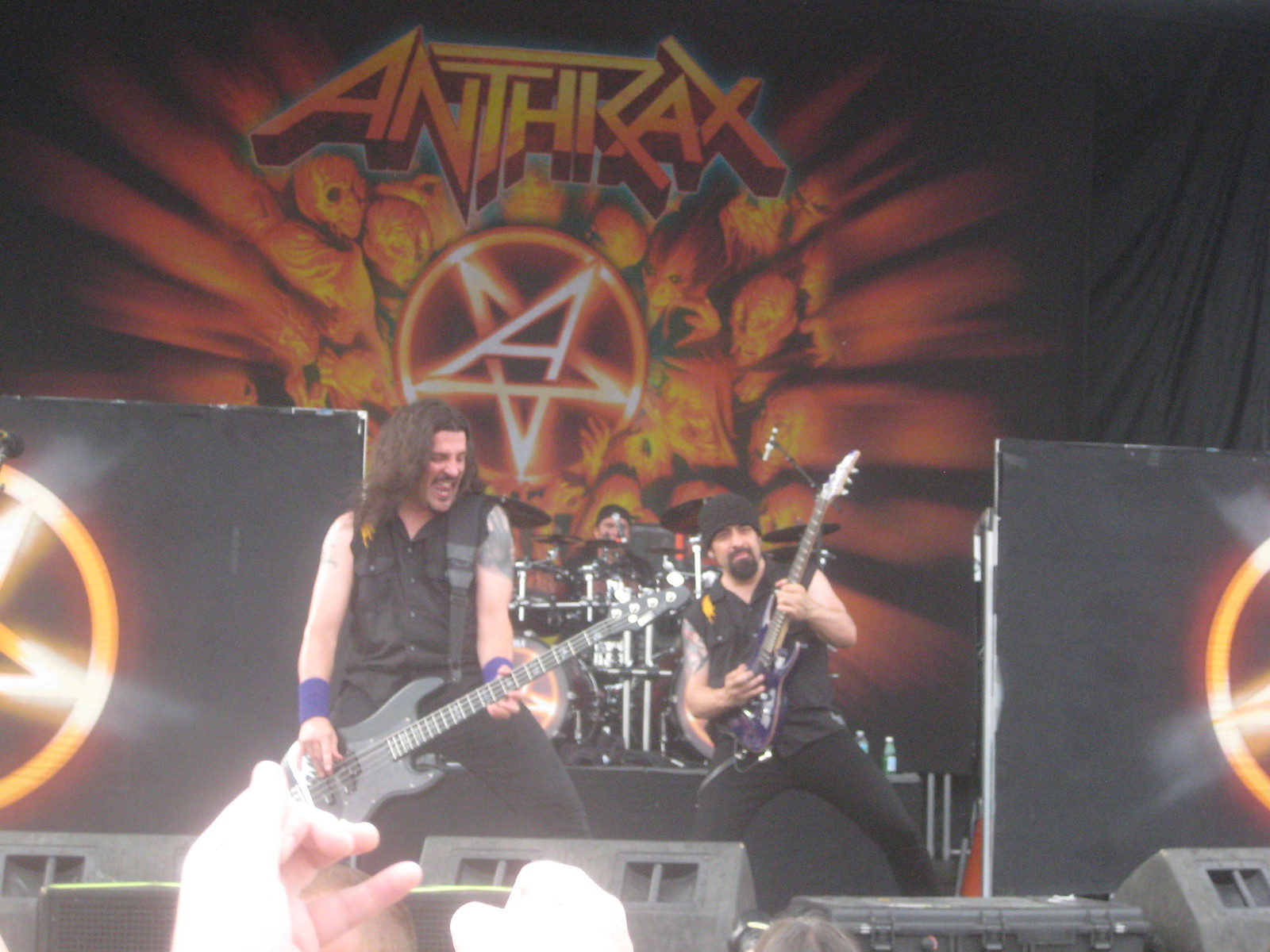This photograph captures the electrifying atmosphere of an Anthrax concert, a renowned heavy metal band, on a dynamic stage backdrop adorned with a large banner that reads "Anthrax." The banner features an intricate design beneath the band's name, showcasing an upside-down pentagram surrounded by demonic-looking creatures. Central to the image is the drummer, positioned on his own elevated stage, wearing a backwards black baseball cap and a dark shirt. Flanking him are two energetic guitarists. The bassist, with long brown hair and wearing a black vest and pants, plays passionately, his black bass guitar in hand and purple wrist guards adding a pop of color. The guitarist next to him, distinguishable by his thick black goatee and black beanie, plays a black guitar with a purple border. He's in a sleeveless black button-up shirt, matching with his bandmate's dark ensemble. Their expressions and bent postures exude motion and enjoyment, enhancing the concert's vibrant energy. Flanking the stage are additional display boards bearing the same emblem as the central banner. Below the stage, the audience's raised hands add to the concert's fervent atmosphere. In front of the musicians, monitor speakers are aimed back at the performers, and black boxy equipment is visible by the stage, completing the immersive concert scene.